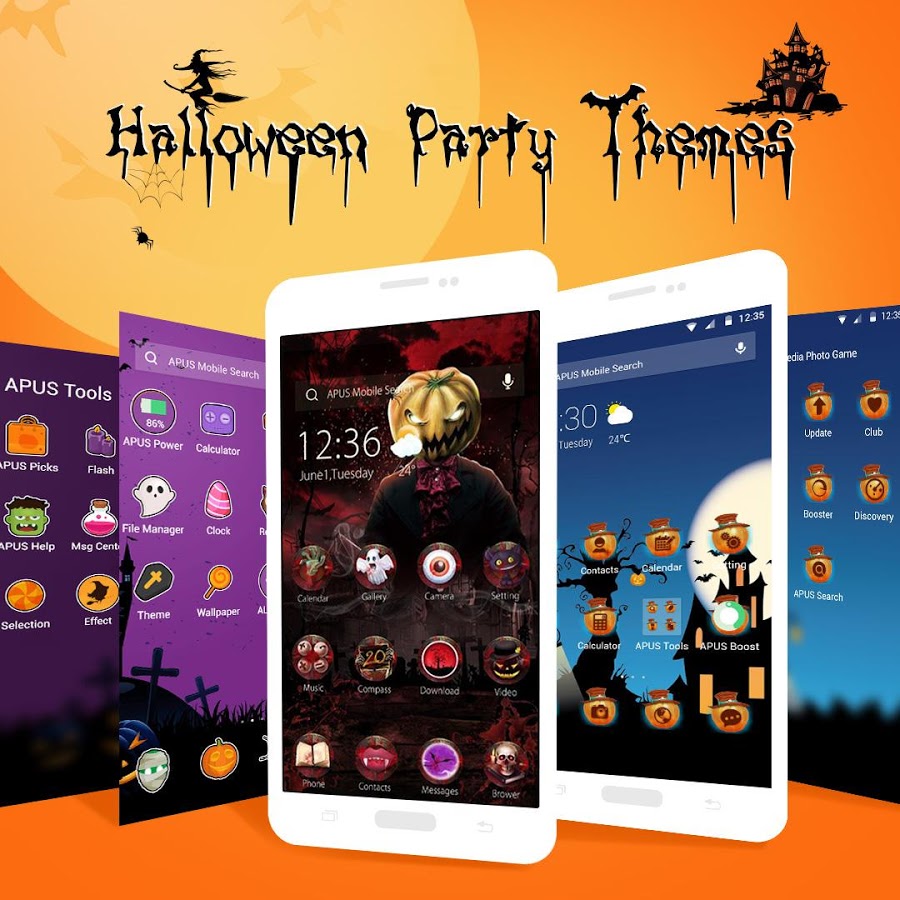This advertisement showcases a selection of Halloween-themed designs for smartphones, potentially for both Apple and Android devices. The promotional image features a square layout with a vivid orange background that fades into a lighter shade for a full moon, positioned prominently near the top left corner. The moon illuminates a playful Halloween scene, including a tiny witch hovering above a Halloween owl, and a small spider dangling beneath the letter "H". Further to the right, a spooky castle looms in the distance, all elements rendered in ominous black.

At the top of the advertisement, the words "Halloween Party Themes" are displayed in a striking, spiky font, each word capitalized and suggestive of the spooky celebrations. Beneath this header, there's a showcase of three distinct Halloween themes designed for phone customization.

On the left, two side-by-side screens display a predominantly purple and black theme. The backdrop is a deep purple with contrasting black icons and images, creating a mystical and eerie atmosphere. The central theme showcases a monstrous creature with a pumpkin head and glowing eyes set against a dark reddish-black background, adding a touch of frightful imagery. Finally, to the right, a cool-toned theme features a blue and black color scheme. The background is a haunting blue, overlaid with black imagery, while the icons pop in golden-yellow hues.

Each theme offers a unique flavor of Halloween spirit, perfect for those looking to embrace the festive season on their smartphones.